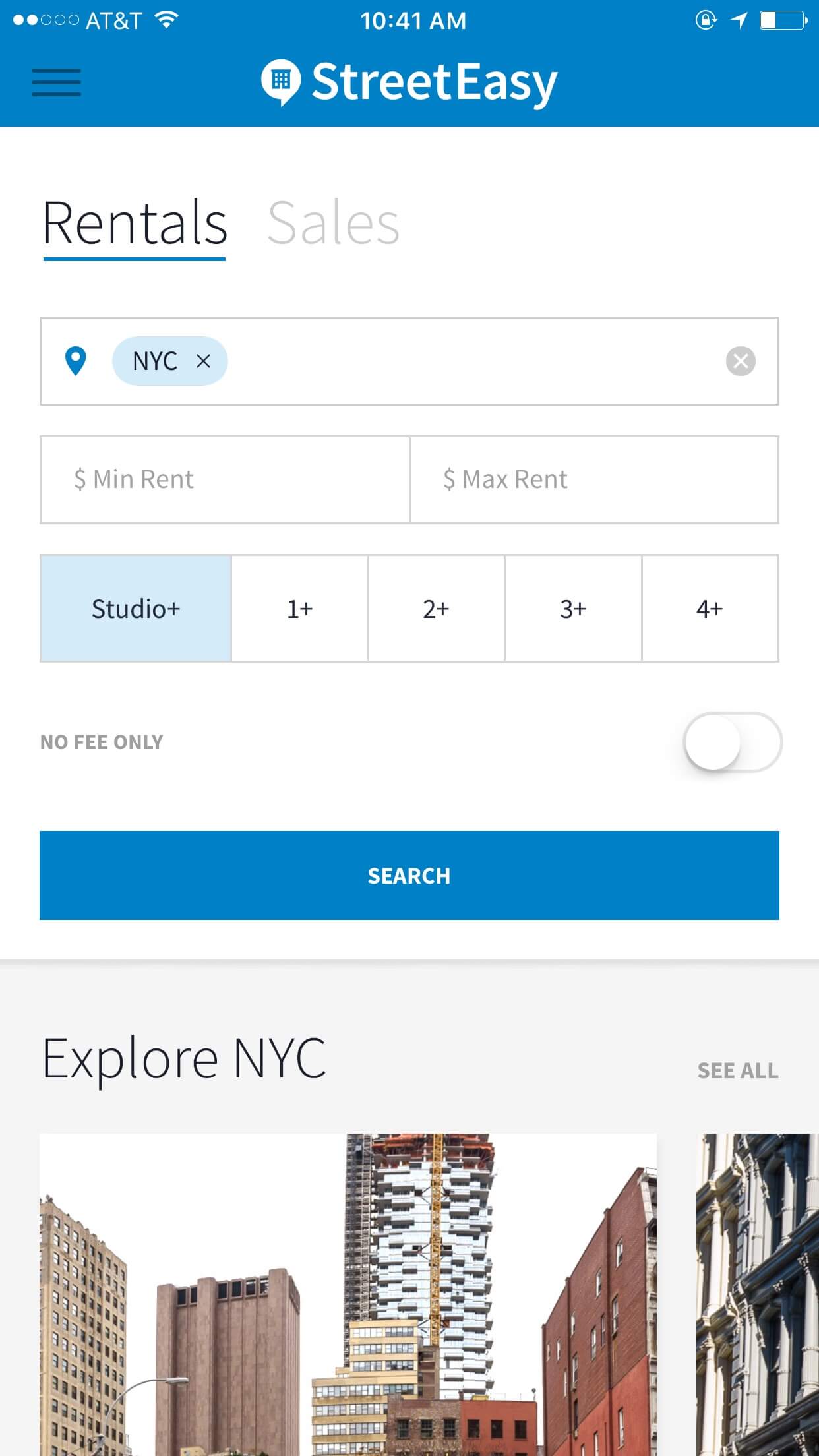**Detailed Caption:**

This screenshot captures the interface of a smartphone displaying the StreetEasy app, a popular real estate platform. At the top left corner, the screen shows the service provider information along with reception and Wi-Fi status. The current time, 10:41 AM, is prominently displayed in the center. On the top right, various status icons indicate features such as orientation lock, active location services, and battery status. The screen's top portion is shaded in blue, transitioning to a primarily white background with a grayish-white color towards the bottom.

Central to the screenshot, beneath the time, is the StreetEasy app's header, featuring its logo to the left of the app name. Just below the service provider information on the left, three horizontal lines suggest a menu option. The main body of the screen displays tools for browsing real estate listings: two tabs for selecting between rentals and sales, and a location input box. Underneath, users can specify minimum and maximum rent, and choose the number of bedrooms from studio to four bedrooms. A toggle button labeled "No Fee Only" is turned off, followed by a prominent blue "Search" button in white font.

In the grayish-white lower section, the heading "Explore NYC" is visible alongside a small "See All" button, hinting at further exploration options. Partially shown below this heading is an incomplete picture of New York City, contributing to the visual focus of the app's interface.